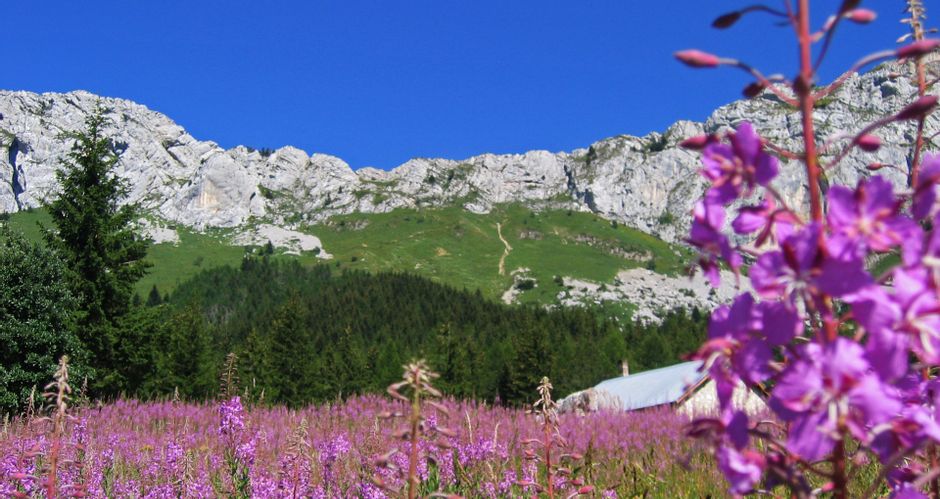The photograph captures an enchanting, multi-layered natural landscape. In the foreground, there is a close-up of vibrant purple flowers on a pink stem, slightly out of focus, which leads into a sprawling field teeming with hundreds, possibly thousands, more of these striking flowers. Nestled within this sea of blooms, partially concealed, is a house with a chimney; the off-white structure has a slightly gray roof that peeks out subtly. The field fades into a dense forest of various tall, dark green evergreen trees, gradually transitioning into lighter shades of greenery as it climbs the hillside. Further back, an imposing mountain stands majestically, its white and light gray rocky surface sharply contrasting with the lush greenery below. Above all of this, a brilliant, cloudless blue sky stretches across the top of the image, occupying about 15% of the frame, completing the picturesque scene devoid of any signs of animal life, capturing the serene beauty and layers of the natural world.